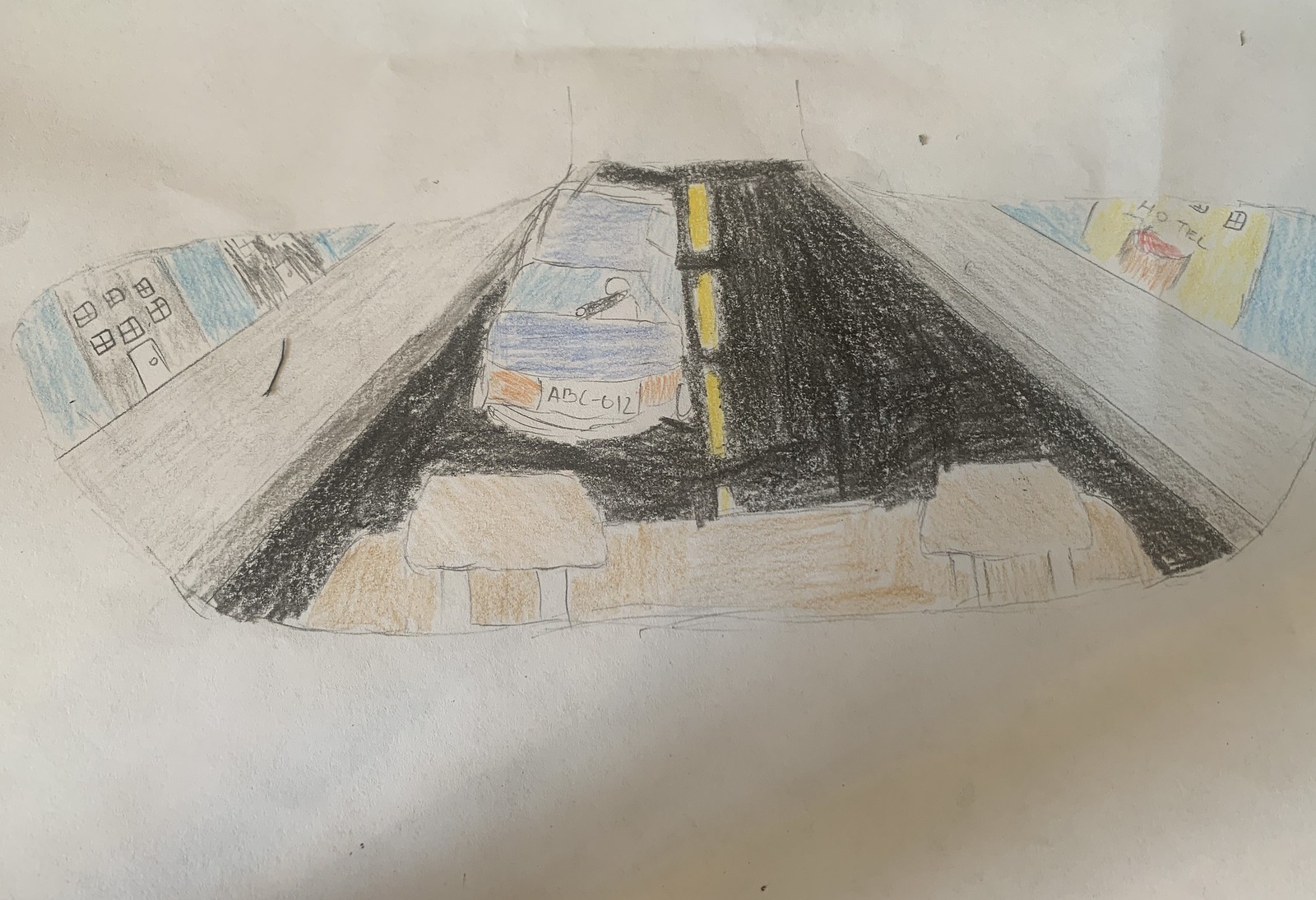This is a photograph of a crayon drawing, seemingly crafted by a child, depicting a forward-facing perspective of a street. The scene is viewed from the vantage point of someone driving a large truck, suggested by the presence of headlights and a grill at the bottom of the image. A blue car, with visible orange headlights and a license plate, travels along the road. The car features a person resting their arm on the headrest from the back seat. The central road, marked by a dashed yellow line, is flanked by gray sidewalks on both sides. On the left side of the road are two buildings in shades of gray and black, with one detailed as a rectangular structure having a door at the bottom and six windows above. To the right, a building labeled "Hotel" with yellow walls stands out against the setting. The road appears to curve upward as the drawing fades out, framed by an assortment of blue and shaded areas. Despite its childlike execution, the drawing is impressively detailed and evokes a sense of motion and perspective.